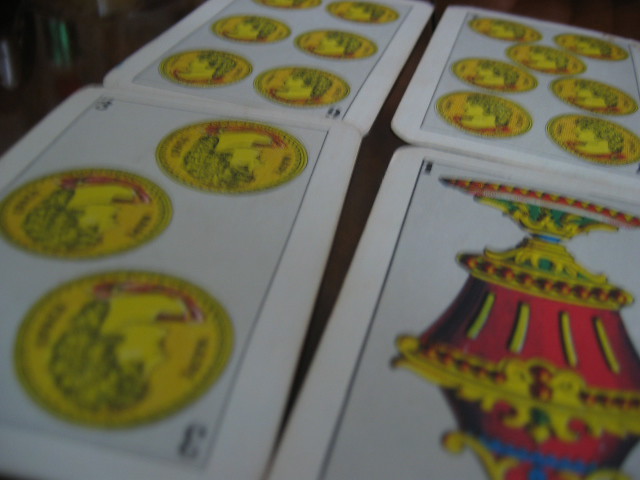This image features four Italian Briscola playing cards meticulously laid out on a dark table under dim lighting, giving the scene a mysterious, almost nocturnal ambiance. The cards display intricate designs, including coins with detailed heads embossed on them and an ornate urn or vase. Among the visible cards, one is marked with the number '3', another with '6', and a third with '1'. The fourth card, although not entirely visible, prominently features coins that likely indicate its numerical value. The arrangement of the cards adds to the intrigue: two are positioned upside down, obscuring some details, while the other two face the viewer. The overall image is somewhat blurry, adding to the enigmatic feel of the scene and making it challenging to discern finer details.